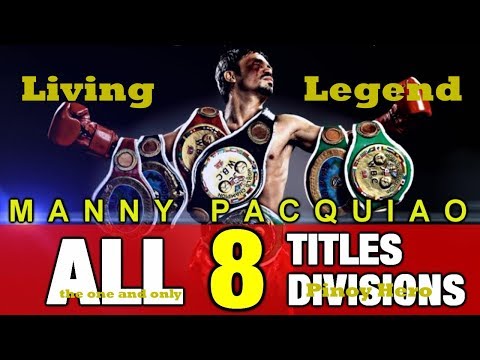The image is an illustrated graphic of the legendary boxer Manny Pacquiao. He is depicted shirtless, with a heavy set of championship belts draped over his arms and hanging from his waist. Each belt is uniquely colored: the ones on his body are brown and black, the one on his left arm is brown and blue, and the one on his right arm is green. Manny is wearing red boxing gloves, and he has a black eye, emphasizing his resilience. The background of the image is predominantly black, highlighting the visual elements and texts.

To the left and right of Manny Pacquiao, in gold font, is the text "Living Legend". Below Manny, his name is prominently displayed in all caps and gold color. Beneath this, a red horizontal stripe contains the words "All Eight Titles Divisions," with "All" and "Title Divisions" in white block letters and the numeral "8" in bright yellow outlined in black. The graphic exudes a sense of achievement and prominence, celebrating the boxer's illustrious career.